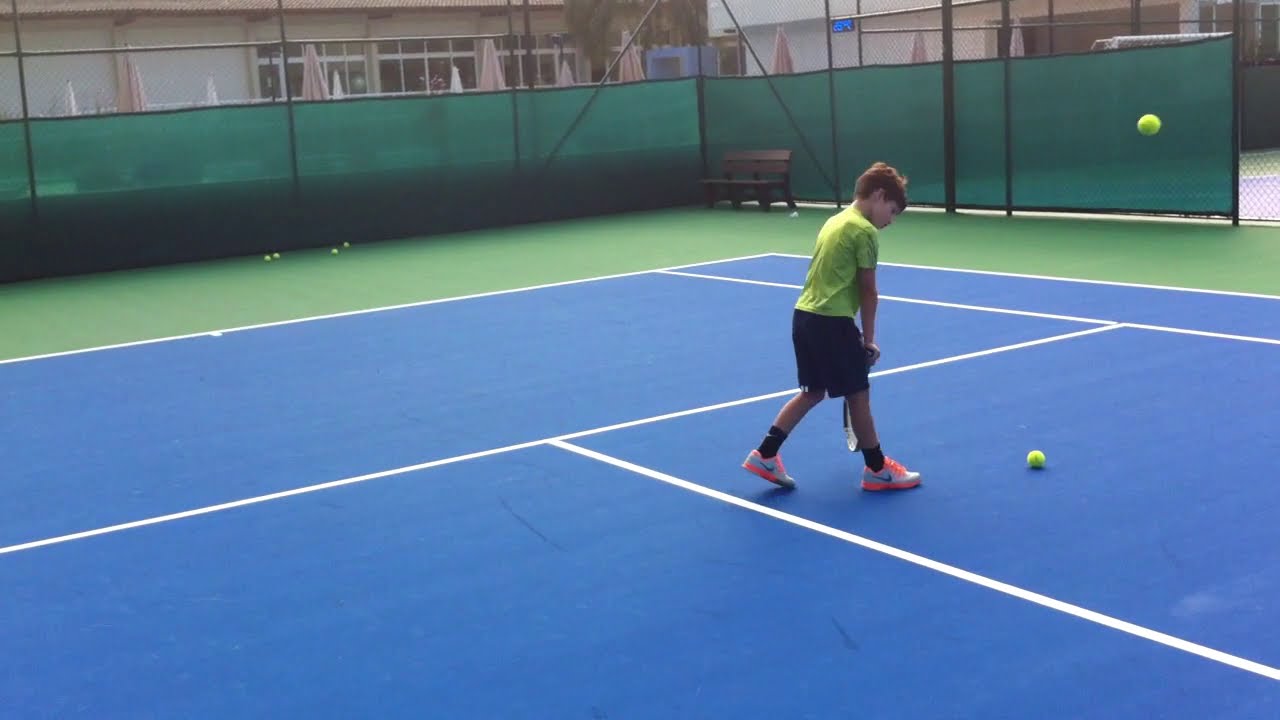The vividly detailed photograph captures an outdoor tennis court scene. The court features a bright blue playing surface with clearly marked white lines and a green border. Encircling the court is a tall chain-link fence adorned with green privacy fabric, with hints of a building—possibly a school or recreational facility—and multiple courts visible in the background. A few umbrellas are faintly visible behind the netting, though none are open.

Central to the image is a young boy with a lighter complexion and brownish-red hair, wearing a neon yellow (or lime green) short-sleeved t-shirt, black shorts that stop just above his knees, black socks, and distinctive orange and white neon Nike sneakers, identifiable by their black swoosh logo. He is holding a tennis racket and appears to be in mid-motion, bending over to pick up a tennis ball from the ground in front of him. 

Scattered tennis balls can be seen around the scene—some near the bench in the corner and others along the green privacy fence. Notably, one tennis ball is captured suspended mid-air. The bright, clear image is well-lit by natural outdoor light, enhancing the vibrant colors and making every detail crisp and clear.